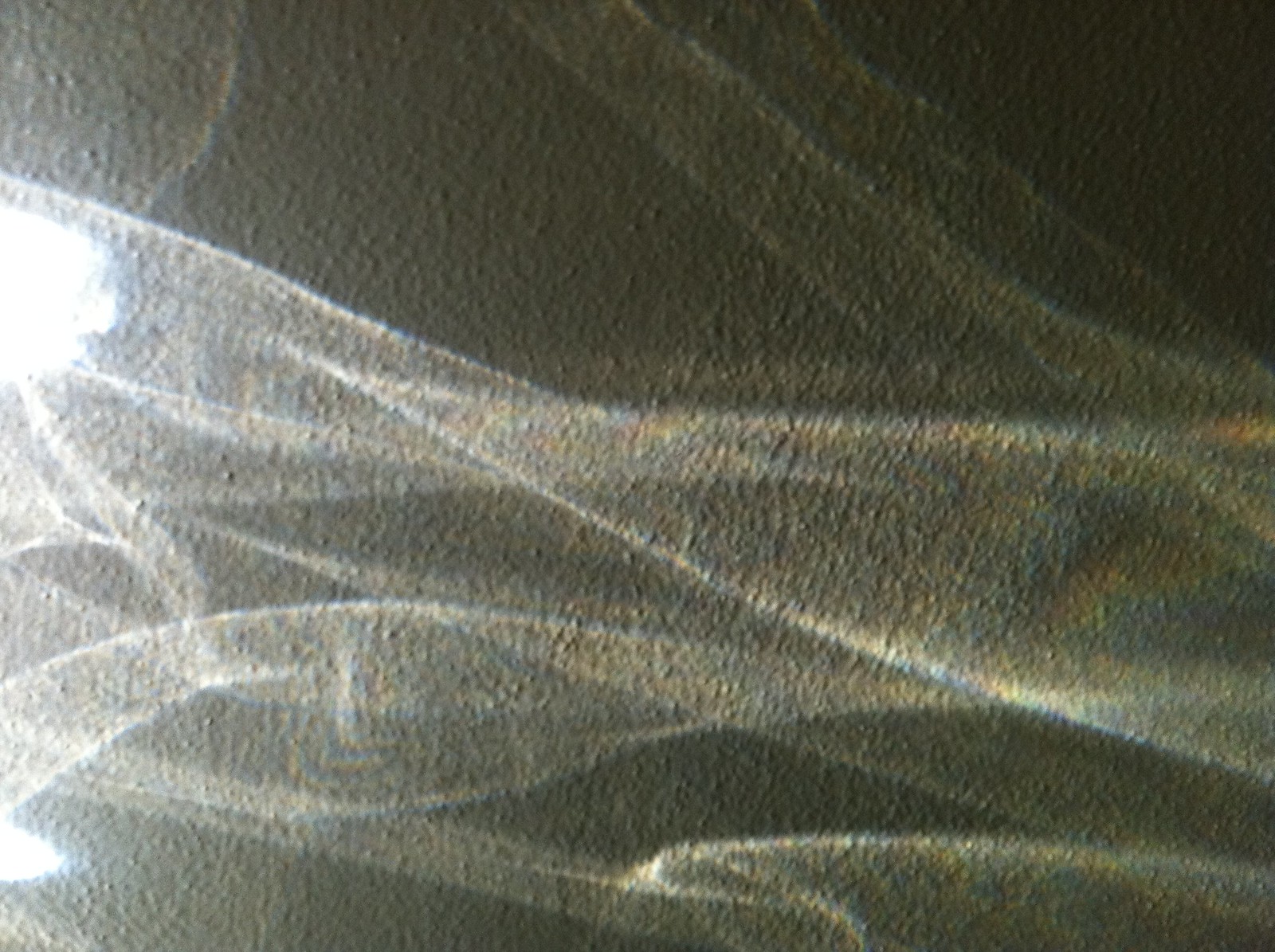The image features an abstract scene dominated by a gray, bumpy wall with small ridges, and through this wall flows a series of white, smoky, billowy shapes that resemble the effect of smoke blown sideways. These lines of smoke create a visual effect as if someone had drawn with white chalk across the uneven surface of the gray wall. In the top left corner, there is a very bright light source that casts shadows and makes the wall appear illuminated, fading into darkness towards the right side of the image. Amongst the white smoky patterns, there are faint hints of rainbow colors, creating an ethereal, almost prism-like effect. The entire composition is reminiscent of swirling light patterns and shadows on a rough, gray canvas.